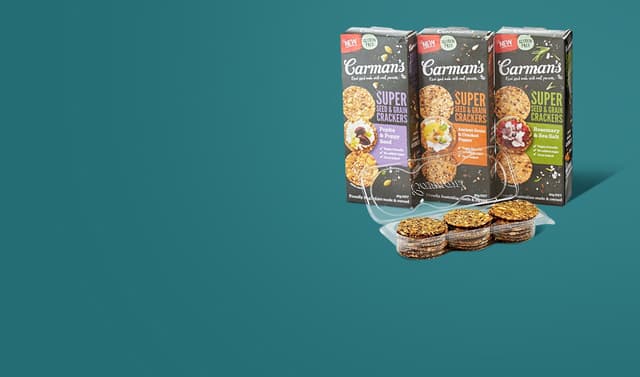The photograph, in a landscape orientation, showcases a vibrant teal background with three black rectangular boxes of packaged crackers prominently positioned in the upper-right section of the image. The boxes are arranged in a stepped formation: the leftmost box is slightly forward, the middle one set slightly back, and the rightmost box further back. Each box features a trio of vertically stacked crackers on the left side, each middle cracker adorned with various toppings, indicating different flavors.

The brand name "Carman's" is displayed in white text on a black background at the top third of each box. Additionally, the boxes have a red horizontal rectangle in the top left corner stating "new" in white text. Next to the cracker images on each box are colored labels denoting the flavors—purple on the leftmost box, orange in the middle, and green on the right. A partially visible round white label indicates that the crackers are gluten-free. In front of the boxes, an opened plastic package reveals three stacks of crackers, arranged left to right in a slight diagonal.

The overall composition and vibrant colors suggest that this image is intended for advertising purposes.